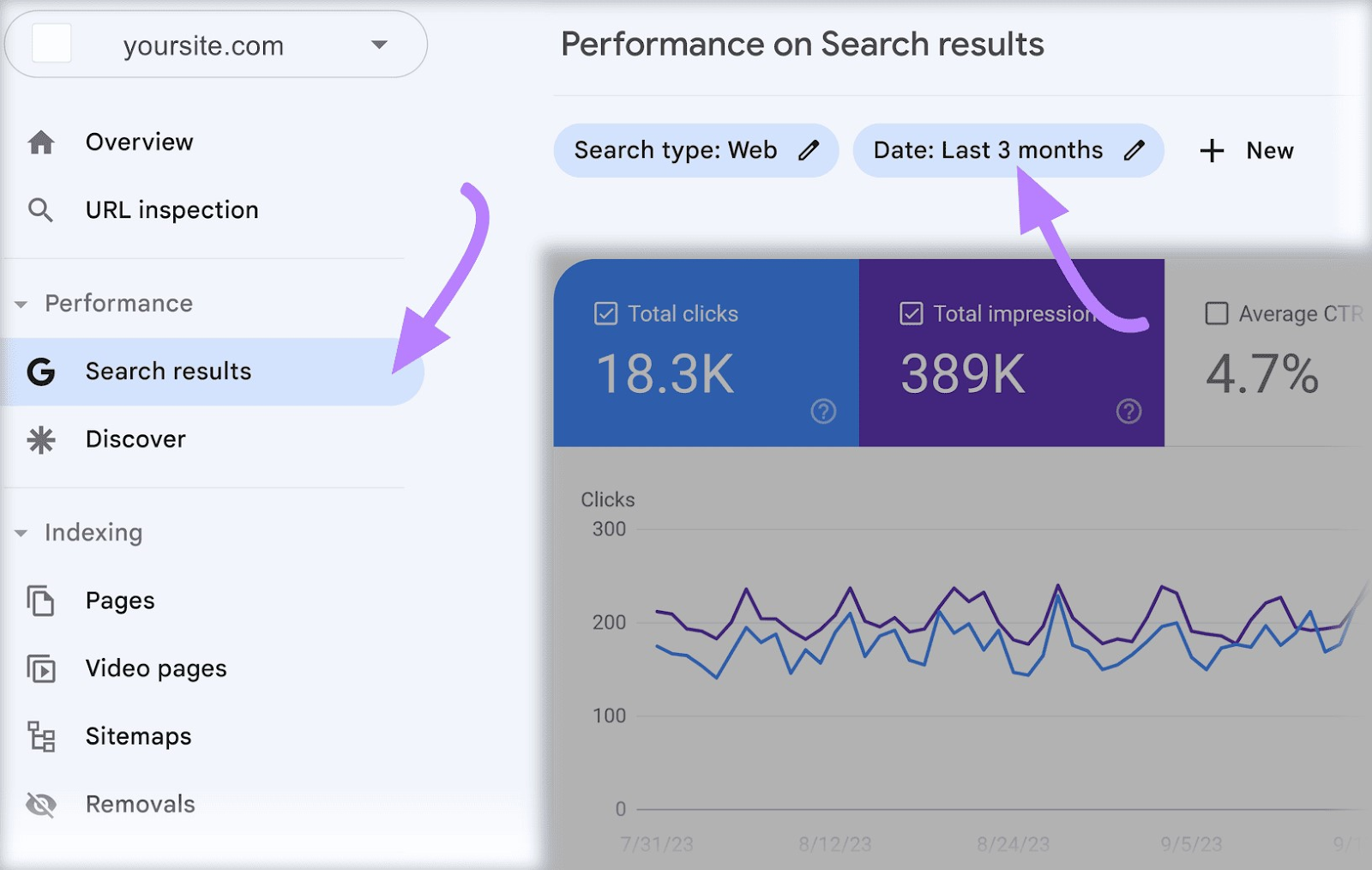The image depicts a website interface showcasing performance metrics for YourSite.com. The top left corner displays "YourSite.com." Below this, a vertical menu on the left side features several options: Overview, URL Inspection, Performance, Search Results, Discover, Indexing, Pages, Web, Video Pages, and Sitemaps. The central part of the image highlights the "Performance on Search Results" section.

A blue-highlighted area details the search engine type as "web" and the date range as "last three months." Two purple arrows emphasize key elements: one points to the "Search Results" option in the menu, which is highlighted in blue, and the other points to "last three months."

Below this, key metrics are displayed:
- Total Clicks: 18,000.3
- Total Impressions: 389k
- Average CTR: 4.7% (Note: The information following CTR is cut off and blurred).

A partially visible chart showcases performance data, with the y-axis showing clicks ranging from 0 to 300 and color-coded lines indicating performance data. The purple line represents total impressions (389k) and stays above the 200 mark, while the blue line corresponds to clicks, fluctuating around the 200 mark. The bottom part of the chart is cut off, obscuring some details.